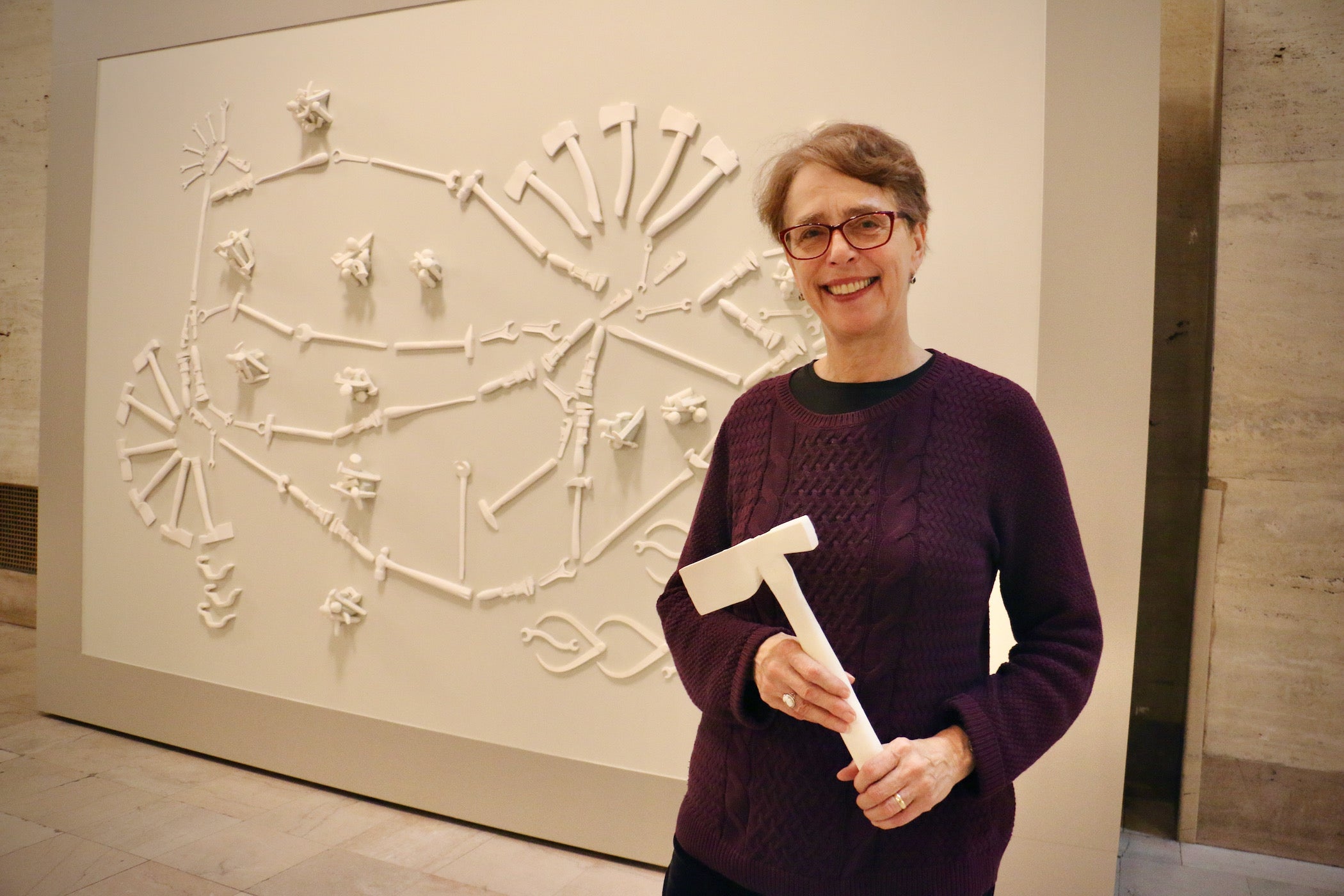In the photograph, a slightly older Caucasian woman with short, light brown hair, parted on the side, stands indoors in front of a large, horizontally-aligned, wall-sized picture collage. She is smiling warmly, showcasing her red lipstick and red-rimmed glasses. The woman is dressed in a burgundy, long-sleeve knit sweater layered over a black shirt, and she has black pants on. Adorning her fingers are rings, with one prominently seen on her left ring finger, suggesting she might be married.

In her hands, she holds an almost-white wooden carving in the shape of an axe. Behind her, a large framed picture, taller and wider than she is, leans against a light brown tiled floor and a similar colored wall. This extensive piece of art features numerous natural wood-colored tools – including axes, hammers, and wrenches – forming a cohesive artistic scene against a beige background. The artwork seems meticulously crafted and might illustrate a larger structure, possibly a tractor. The overall setting suggests she could be intimately involved with the creation, possibly as the artist.